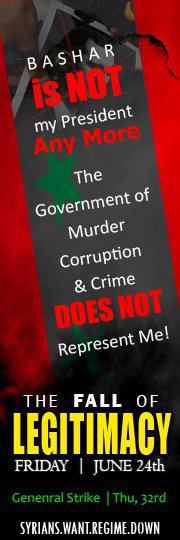The image depicts a rectangular, bookmark-proportioned advertisement with a strong focus on text rather than objects. The background is primarily red with a black bar running down the center, accentuated by gray and green highlights. The text layout is well-spread, ensuring readability. At the top, in red and white letters, it reads “Bashar is not my president anymore.” This is followed by a green star, and the statement “The government of murder, corruption, and crime does not represent me” in a mix of white and red fonts. Further down, the phrase “The fall of legitimacy” is prominently displayed in large yellow letters, with “Friday, June 24th” in smaller white font beneath it. At the very bottom, in green letters, it announces a “General Strike Thursday 32nd,” and underneath that, it is signed off with “Syrians.want.regime.down.” The overall style and elements suggest it's an advertisement aiming to rally support for a political strike against the government.